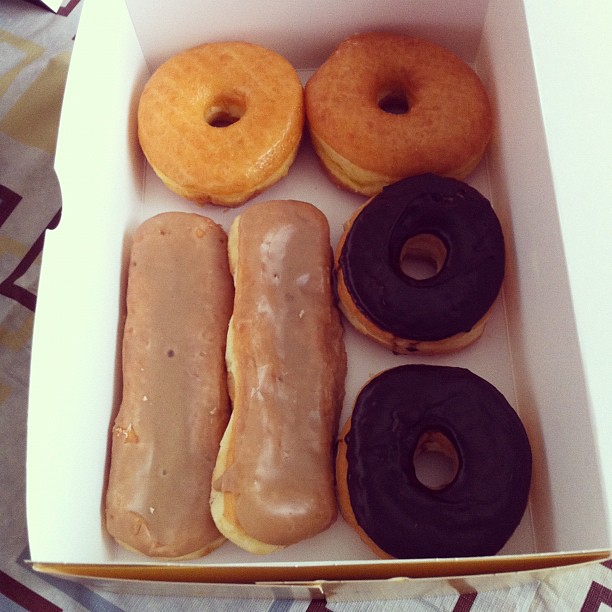The image depicts a real photograph of a box of assorted doughnuts resting on a white tablecloth adorned with gold squares and yellow and purple patterns. The box, made of thin white cardboard, has its sides interconnected and lacks a top, revealing six distinct doughnuts inside. At the top are two shiny, simple glazed doughnuts with a tan hue. The bottom right contains two rich chocolate-covered doughnuts with thick, dark brown icing. To the bottom left are two long, oblong doughnuts, resembling hot dog buns, coated in shiny light brown butterscotch icing. The box’s exterior sides appear to be gold, lending a touch of elegance to the scene.